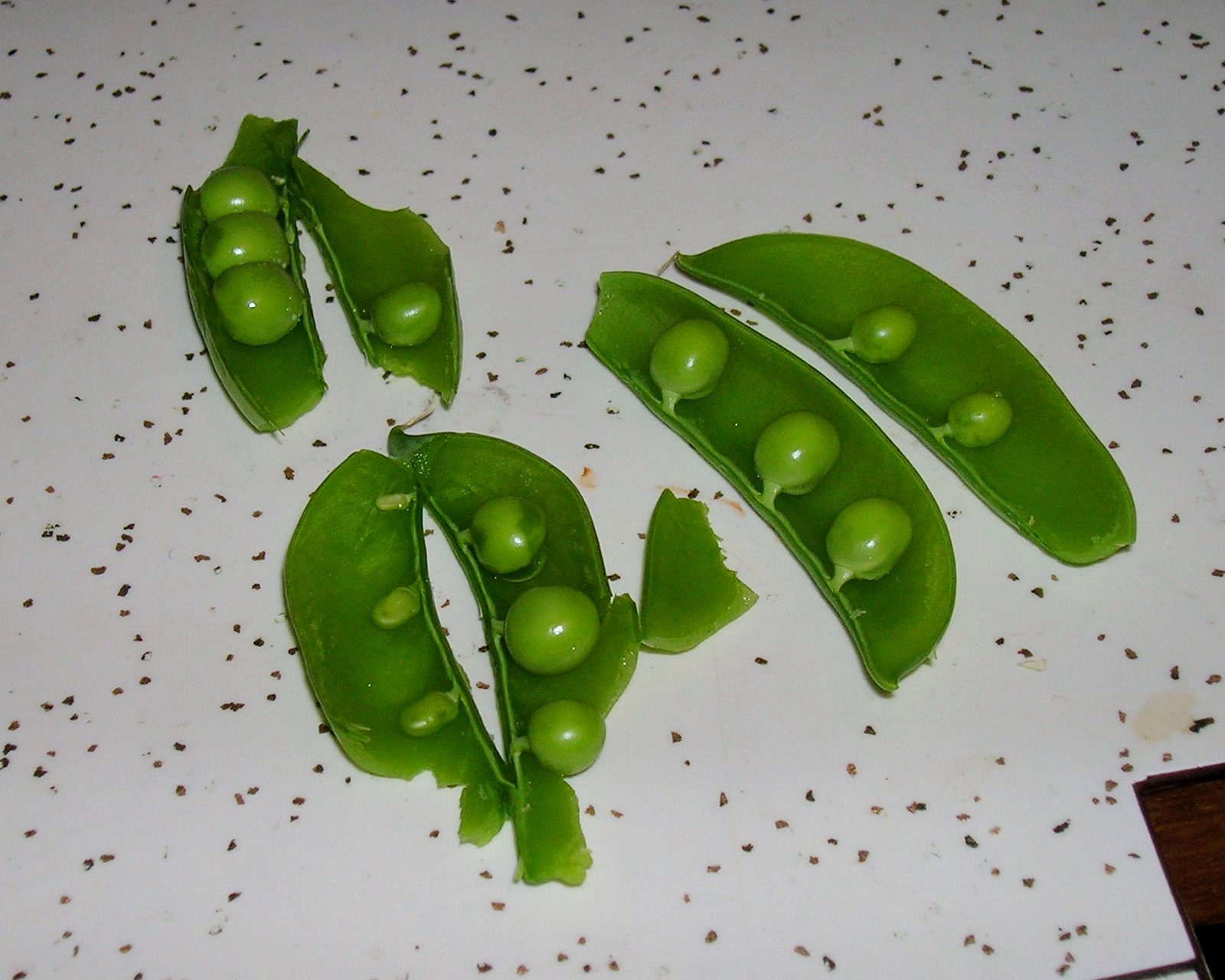On a white surface speckled with black, brown, and green dots, three cut-open green bean pods reveal the immature peas inside. The photo, taken close-up with a personal camera, shows each bean's intricate details. The pod in the upper left contains four peas, while the one in the bottom left has three peas and a broken end. The pod on the right houses three larger peas and two smaller ones. At the bottom right corner of the image, the edge of a surface or book is visible. The peas inside the beans are small and appear not ready for eating.